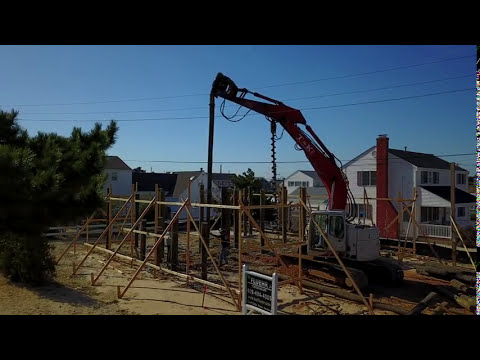The image depicts a vibrant construction zone set against a backdrop of clear blue sky and surrounding houses, primarily white in color with black roofs, and one with a distinctive red chimney on the right-hand side. Central to the scene is a crane, prominently positioned and actively lifting beams and other materials, identifiable by a long black pole extending from it. The foreground is dominated by a wooden frame of a house, emerging from a diligently prepared site of cleared and plowed earth, indicating early stages of construction without a basement visible. There are several wooden poles protruding from the ground, signifying work in progress. Notably, a small bush or tree appears on the left, and a little white sign is discernible in the foreground, adding to the detailed hustle of residential development in what appears to be a neatly framed snapshot of suburban growth.